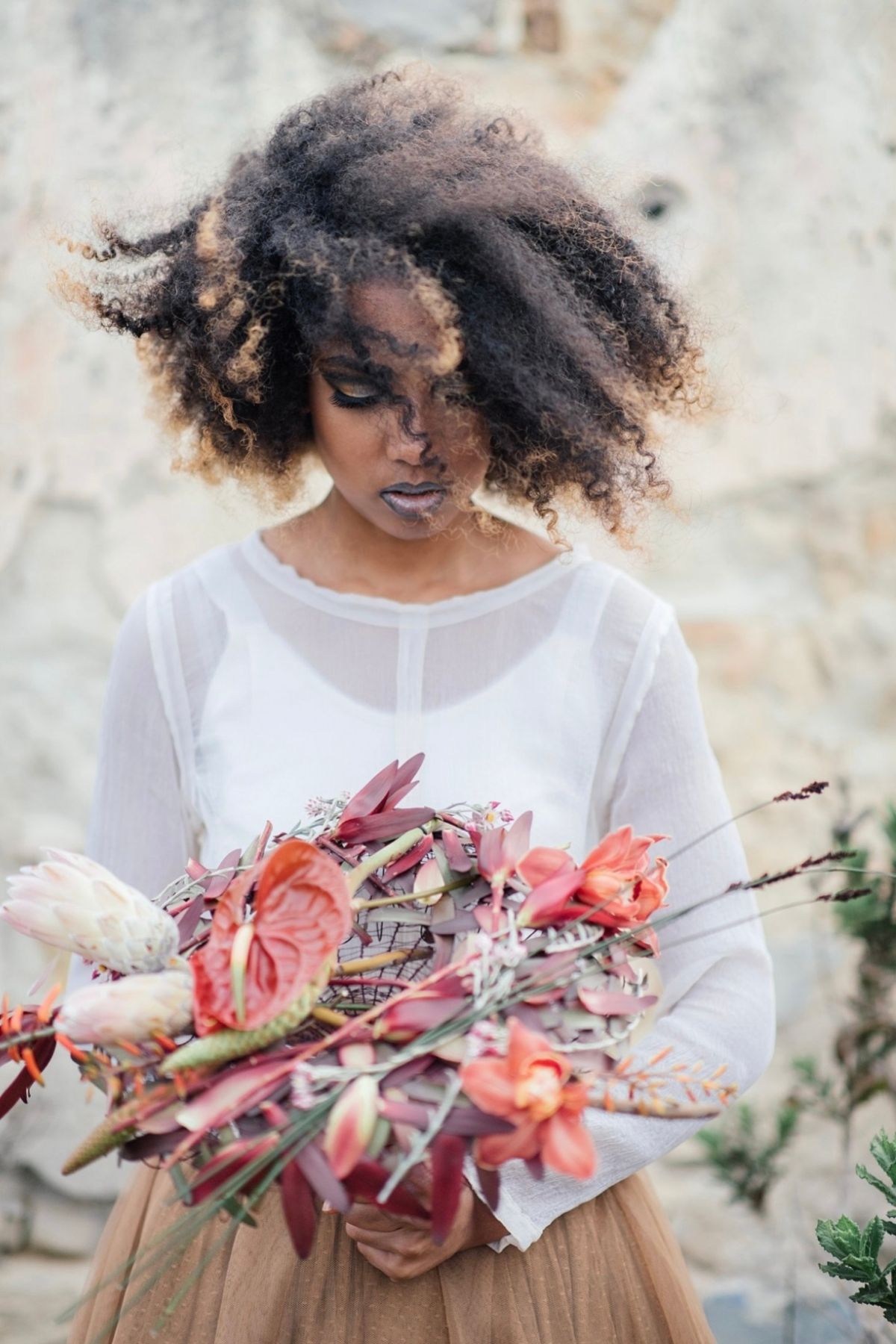In this outdoor photograph, a young woman of African descent stands gracefully, holding a vibrant bouquet of flowers in her hands. The bouquet consists of an array of colors including pink, peach, lavender, and white, and is nestled in a woven basket, though the details of the basket are partially obscured by the lush blooms. The woman has rich, thick coily hair with light brown highlights, giving it a distinctive character. Her makeup is bold, featuring dark lipstick and dark eyeshadow, accentuating her striking features, and she appears to be wearing fake eyelashes.

She is dressed in a sheer, long-sleeved white blouse, under which a fitted white tank top is visible. Her lower half is clad in a frilly, beige A-line skirt. The skirt complements her elegant yet youthful attire and enhances the overall aesthetic of the scene. She stands with her hands clasped at her waist, holding the bouquet in front of her, and her gaze is directed slightly downwards.

Surrounding her, the backdrop features elements of nature; greenery with small leaves is visible to her side, and a gray rocky hillside or ledge provides a textured background. The natural setting enhances the earthy, serene ambiance of the image, framing the young woman beautifully.